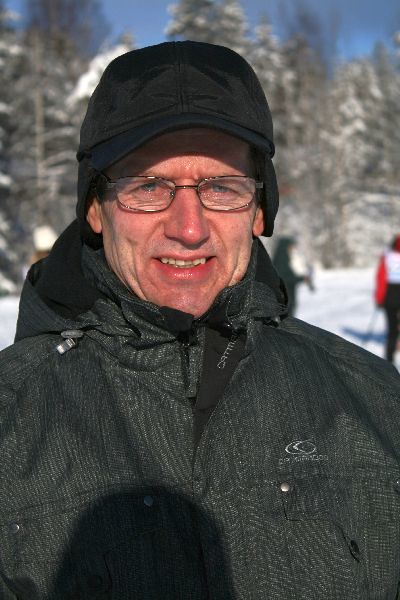The photograph captures an older Caucasian gentleman standing outdoors in a winter setting. He wears glasses that frame his blue eyes and a double-layered headgear consisting of a cap topped with a baseball cap. His face, particularly his nose, appears mildly flushed, likely due to the cold weather. He is smiling warmly despite the chilly conditions. Behind him, snow-covered trees create a picturesque winter landscape. Blurred figures in the background suggest he might be at a ski resort or near a ski slope. The gentleman is dressed in a dark black and gray jacket with a hood, which he has not put on.